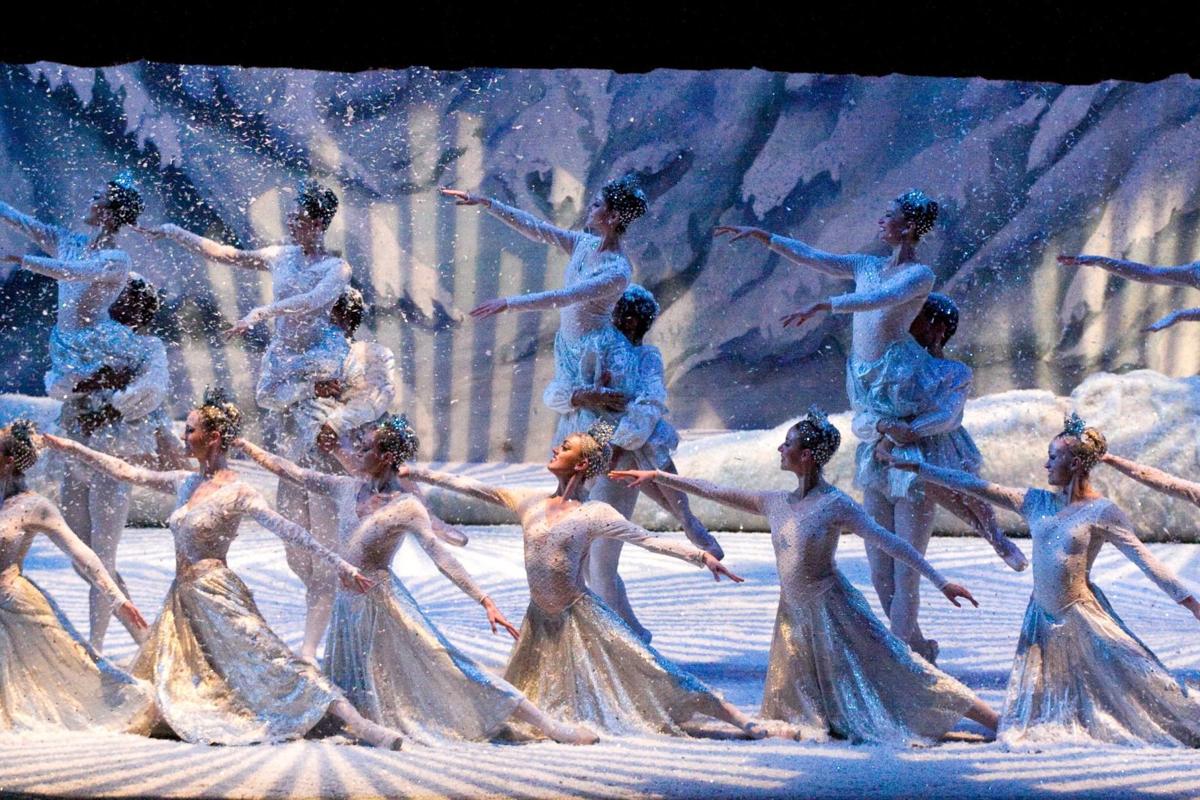This detailed image vividly captures a choreographed ballet performance set in a winter wonderland. In the foreground, six ballerinas dressed in elegant white and silver dresses are gracefully gliding on one foot, their other foot trailing behind, creating an enchanting visual of synchronized dance. Their arms are outstretched, adding to the fluidity of their movement. Surrounding them, faux snowflakes and sparkling confetti gently cascade from above, enhancing the magical ambiance. The stage is also covered in a white substance mimicking snow, blending seamlessly with the decorated background filled with snow-covered mounds and the bottom portions of Christmas trees. Additionally, the back row features pairs of men and women; the men lift the ballerinas, who extend their arms elegantly, contributing to the overall harmony and spectacle of the performance. Multiple rows of dancers in coordinated white and blue attire support the front row, making this scene appear as part of a grand Broadway-style presentation.